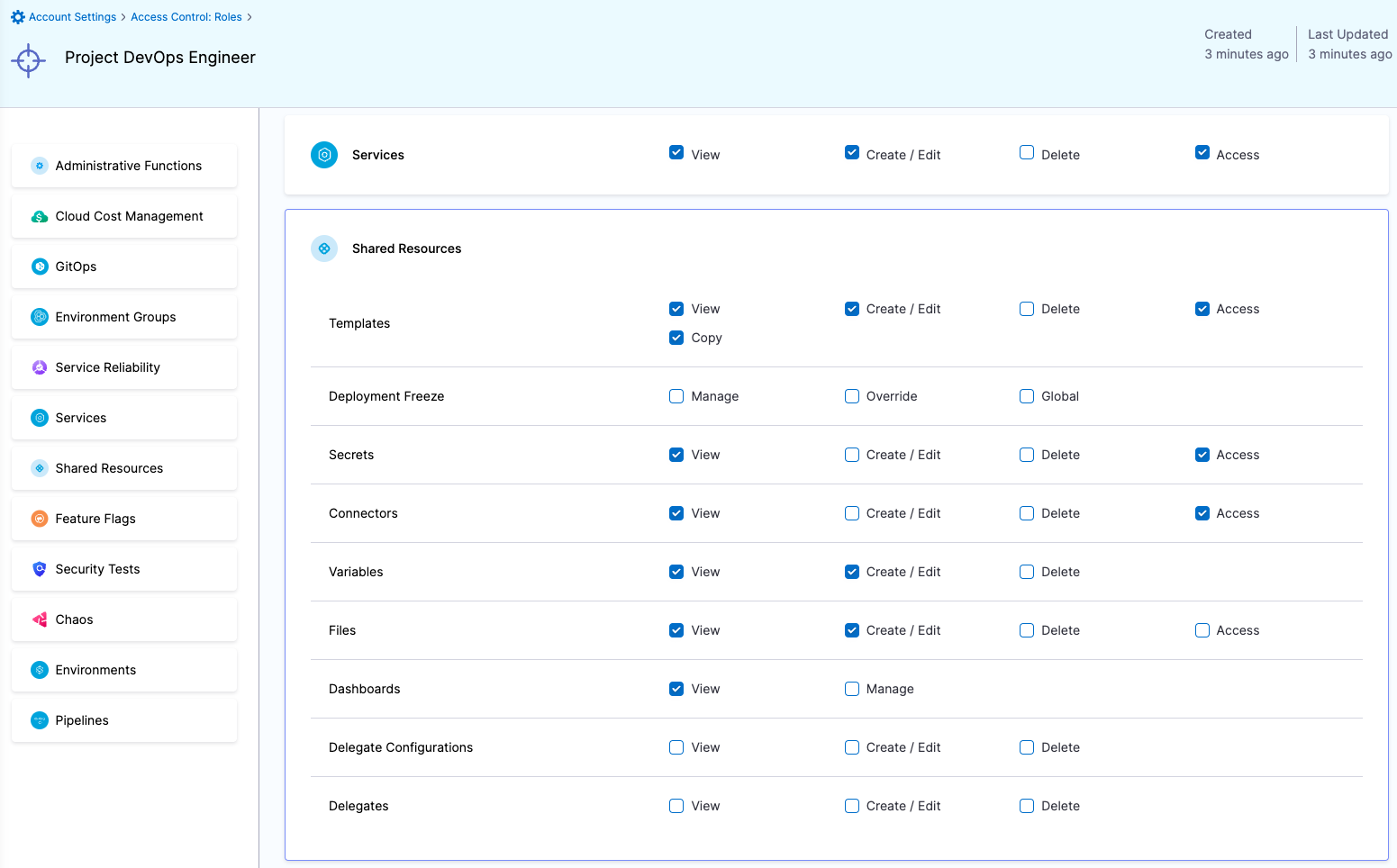In the image, a computer window is displayed titled "Account Settings" and "Access Control." Positioned in the top left corner is a bullseye target icon with a purplish hue. To the right of this icon, "Project DevOps Engineer" is written in black text, all set against a light blue header background. On the far right of the header, it indicates "Created 3 minutes ago" with a vertical gray line dividing it from "Last updated 3 minutes ago."

Below the header, on the left side, there are various options displayed as white buttons with black text and an image icon to the left of each button. Below these options, a large rectangle titled "Services" is visible under the blue header, featuring an icon. This rectangle has a blue border, indicating it is selected, and is labeled "Shared Resources."

Within this section, there is a list of items with checkboxes next to each. Approximately half of these checkboxes are marked. The items listed include: "Templates," "Deployment Freeze," "Secrets," "Connectors," "Variables," "Files," "Dashboards," "Delegate," "Delegate Configurations," and "Delegates."